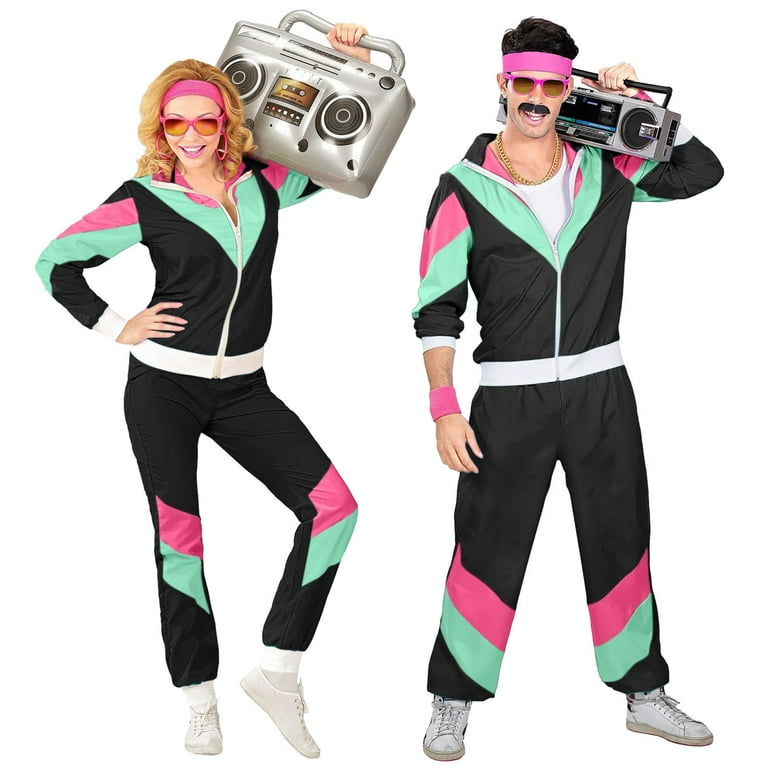This is an image of a Caucasian couple dressed in stylized 80s workout attire, standing against a blank white background. The woman on the left has blonde curly hair, a pink headband, and oversized pink-rimmed sunglasses with an orange reflection, complemented by big pink hooped earrings. She is wearing a retro black exercise suit with a white midsection, cuffs, and zipper. The suit is adorned with muted green V-patterns on the chest and pink streaks that extend up to the hood and are also present on the elbows and knees. She holds an inflatable silver boombox on her left shoulder and wears classic white sneakers. The man on the right sports a thick black mustache, a pink headband, pink sunglasses with a brown reflection, and a double row of gold chains around his neck. His outfit mirrors the woman's, consisting of a black, green, and pink tracksuit with similar patterns and streaks. He holds a real silver and black boombox on his left shoulder and has a pink wristband on his right wrist. Both are smiling and looking directly at the camera, embodying a vibrant and nostalgic 80s vibe.